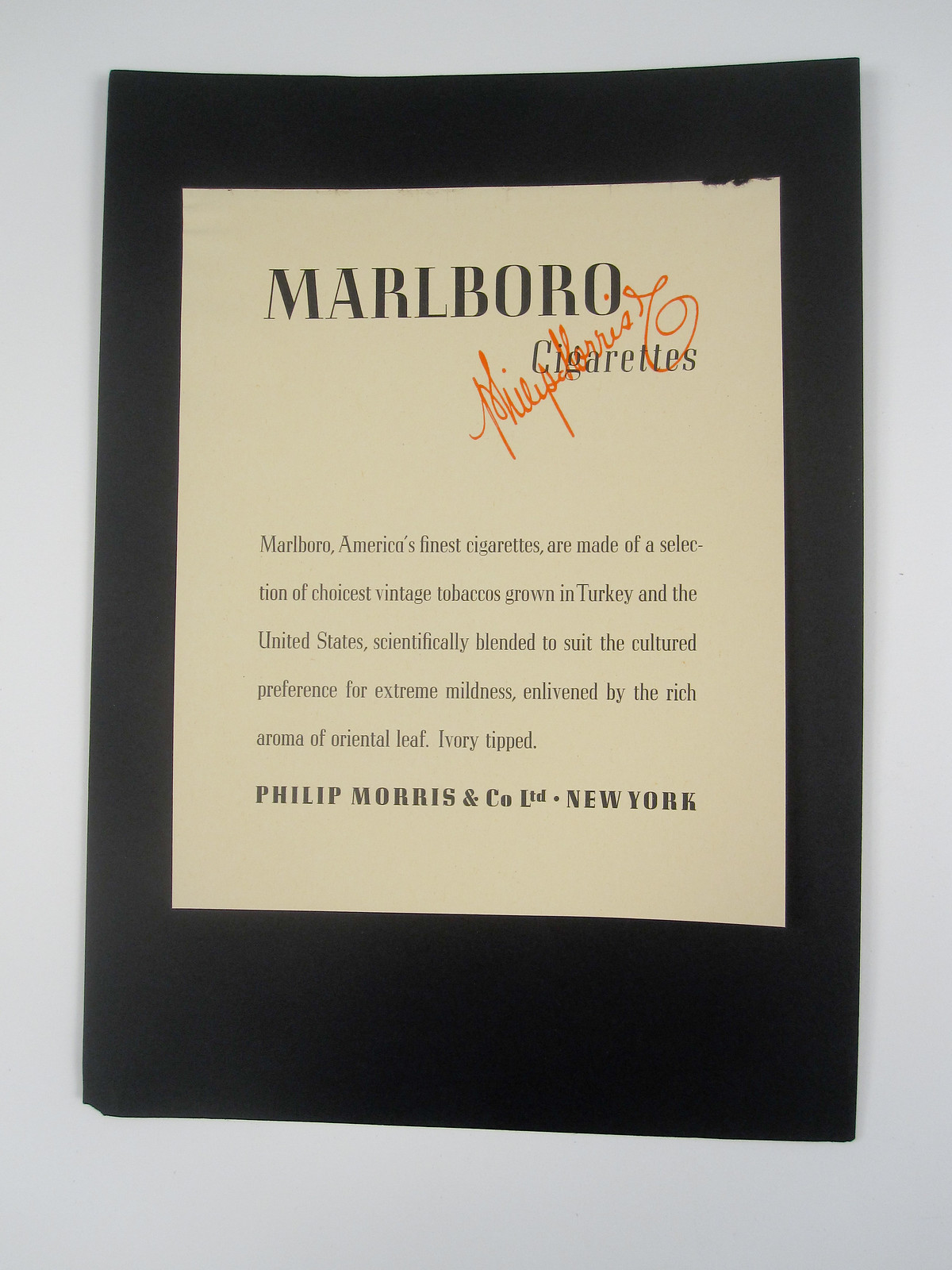The image features an announcement taped to a gray wall. The announcement is printed on a beige or gray piece of paper, which is affixed to a black piece of construction paper with thick black borders on all sides. At the very top of the announcement, the word "Marlboro" is prominently displayed in large black letters, with a distinctive, red sideways signature that runs through the bottom of the letter "O." Below "Marlboro," in smaller text, the message reads: "Marlboro America's finest cigarettes are made of a selection of choice vintage tobaccos grown in Turkey and the United States, scientifically blended to suit the cultured preference for extreme mildness, enlivened by the rich aroma of oriental leaf. Ivory tipped." At the bottom of the announcement, in larger letters, "Philip Morris and Company LTD, New York" is printed.